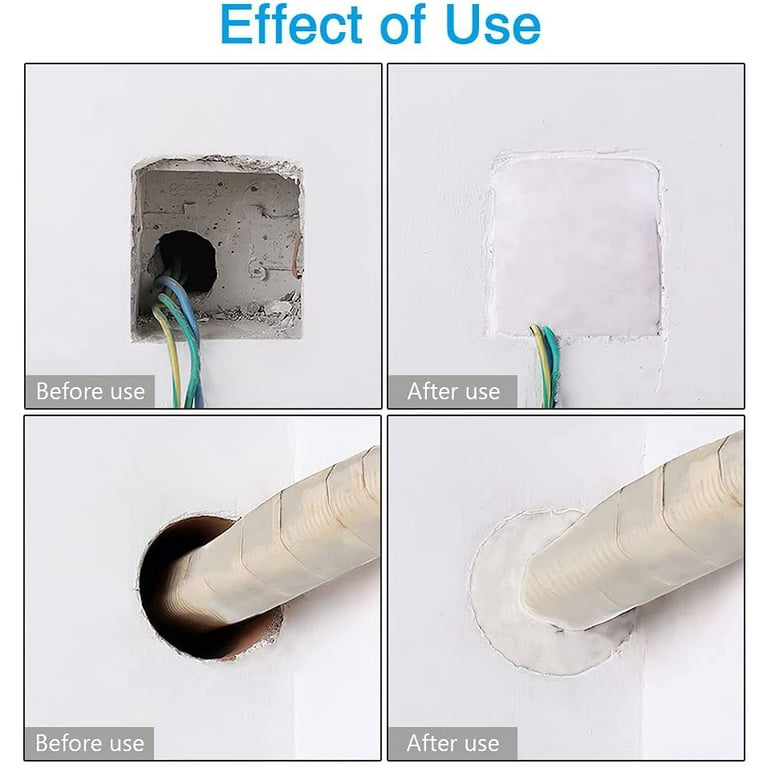The square image displays four labeled photos arranged in a grid, serving as a product advertisement demonstrating the effect of a sealing product. Topped with the blue title "Effect of Use," the top row showcases the "Before Use" and "After Use" of sealing three wires passing through a round hole in a white wall. Initially, a larger square section surrounds the round hole, filled with debris. Post-application, the section is neatly sealed with a clean, white putty, leaving the wires protruding cleanly. The bottom row mirrors this setup, depicting a circular hole with a pipe wrapped in tape. The "After Use" image shows the pipe seamlessly enveloped by the white putty, effectively sealing the gap.